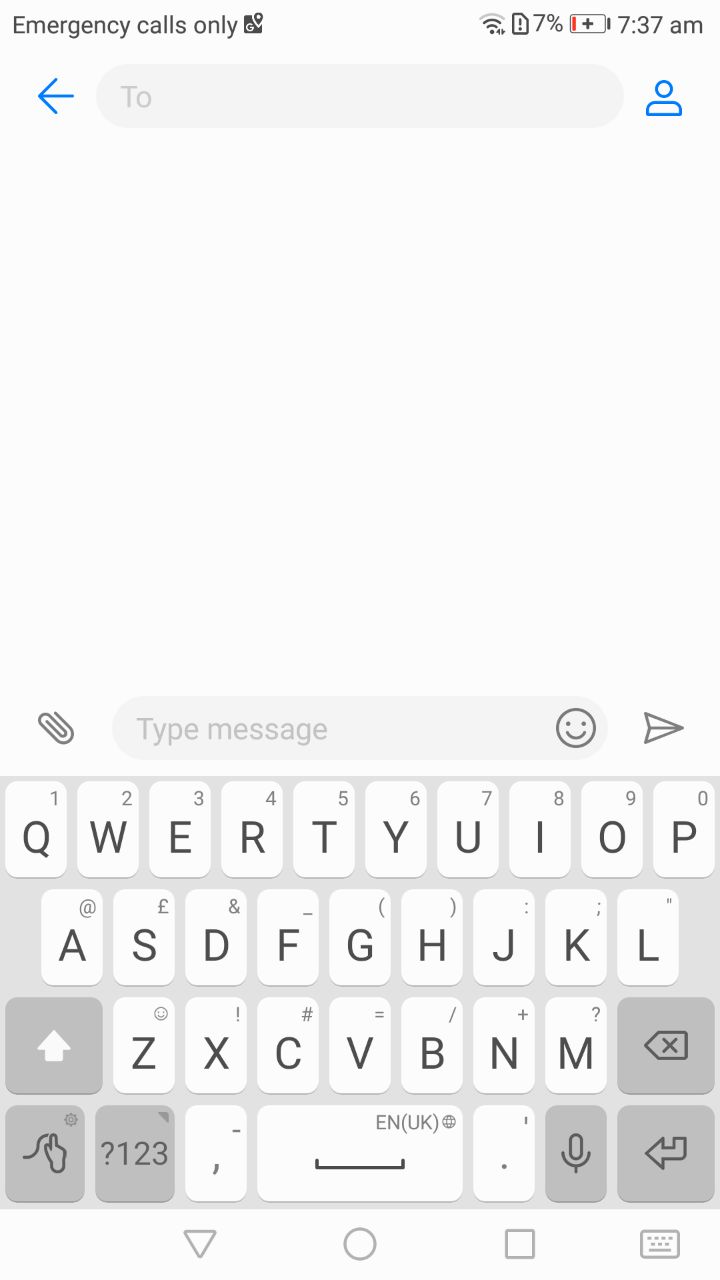The image displays a standard mobile keyboard interface commonly seen when typing a message on a website or through text. The top of the screen indicates "Emergency calls only," with visible icons for a Wi-Fi signal and an error symbol, a battery level at 7%, and a timestamp of 7:37 a.m. Below this notification bar, the text input field is visible, featuring a contact’s name, a person icon, and a blue arrow on the left, indicative of the recipient details. 

The message composition area includes a type-your-message section, complete with an emoji button represented by a smiling face, a send arrow, and an attachment button resembling a safety pin. The keyboard layout follows the QWERTY format, including keys for letters and numbers, with options for special characters. Notably, the language setting is marked as "English (UK)," suggesting the phone's location or language preference might be set to the United Kingdom.

Additionally, a unique feature allows users to hand-draw input, which is not available on all phones. The overall appearance is simplistic, monochromatic, and functional, reflecting a typical mobile keyboard screen intended for text input with no pre-existing text.